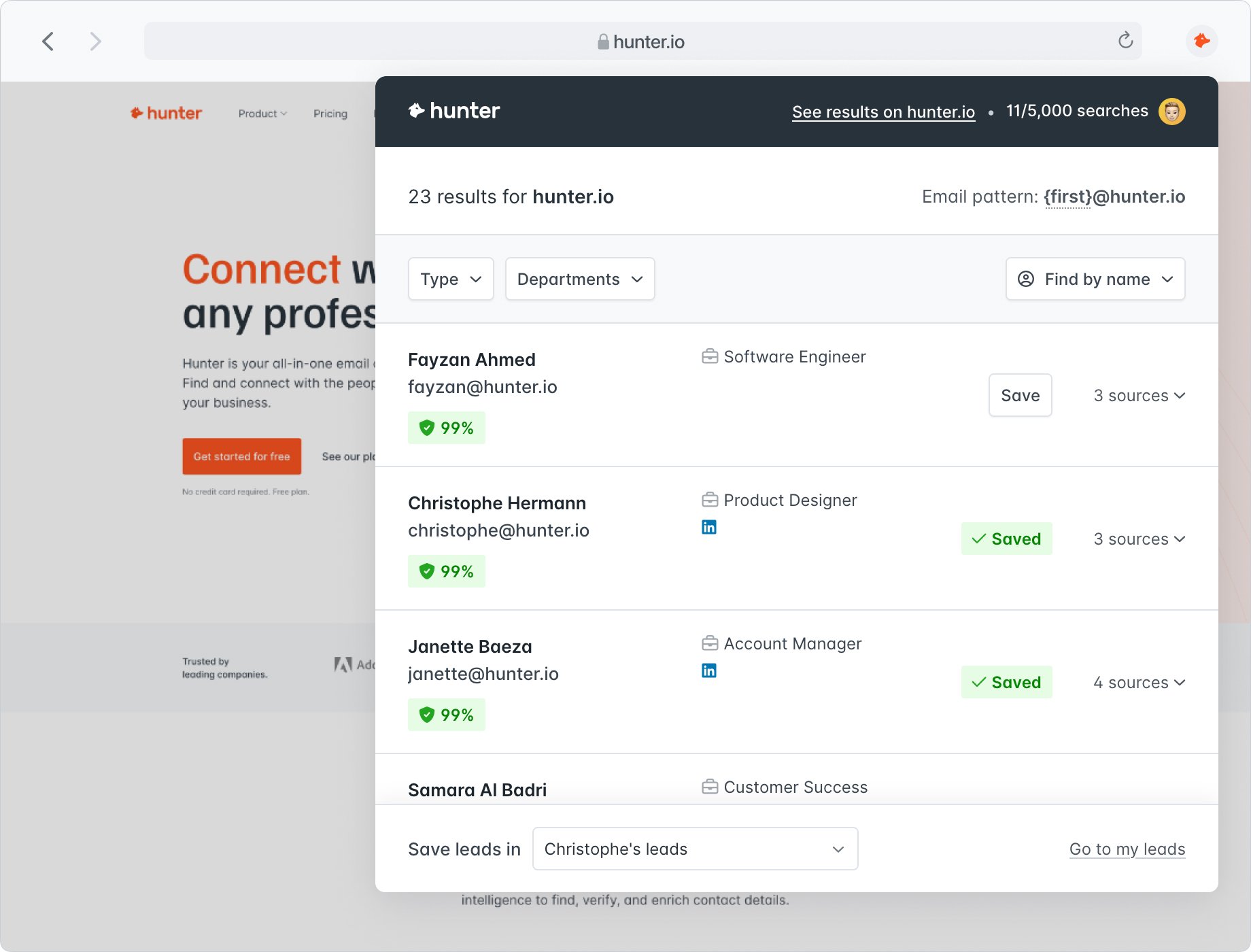This image is a screenshot of a desktop web browser, likely Safari, displaying the hunter.io website. The address bar at the top clearly indicates the URL. The website's interface features a white background with "Hunter" prominently displayed in bold letters at the top left, accompanied by an orange logo. A navigation menu spans from the center to the right, including options such as "Product" and "Pricing."

The central section of the webpage includes a large, eye-catching sentence with the word "Connect" highlighted in orange, followed by a continuation in black. Beneath this sentence is a brief paragraph and a prominently placed orange button. However, this primary view is partially obscured by an overlay, indicating an active pop-up window.

The pop-up window is a sizable white square featuring a dark navy blue header. In the top left corner of this header, "Hunter" and its logo are displayed in white. Across from this, on the top right, text reading "See results on hunter.io" appears as a hyperlink, followed by the note "11-5,000 searches" accompanied by a gold token icon.

The main body of the pop-up reveals a search results page, displaying "23 results for hunter.io" under the header on the left side. The right side of the header mentions an email pattern formatted as "first@hunter.io." Below this, a table lists employees with hunter.io email addresses, organized into columns. Each entry details the person's name and email, their job title (such as Software Engineer or Product Designer), and multiple verified sources, indicated by checks and notes like "3 sources" or "4 sources," along with drop-down options denoted by carets.